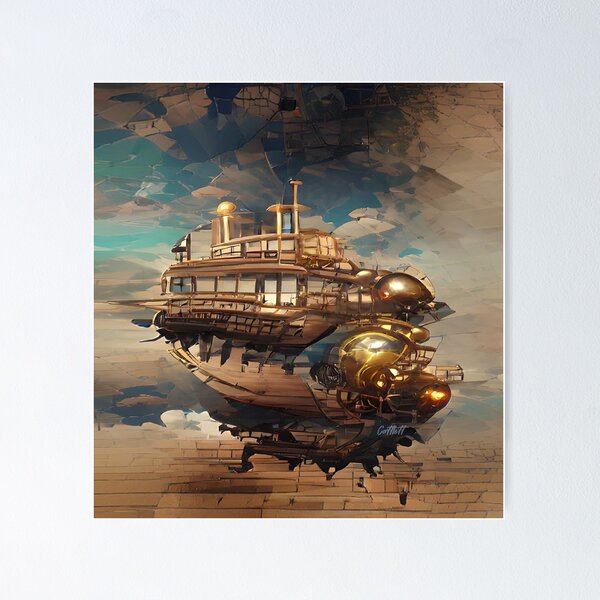The image depicts a highly detailed and imaginative digital painting featuring a steampunk-inspired airship floating amidst a surreal, clouded background. Encased in a gray border, the artwork boasts a complex design blending elements of nautical and aviation aesthetics. The airship resembles a luxurious yacht or houseboat made of wood, featuring numerous glass windows and observation decks for passengers to enjoy panoramic views. Prominent golden metallic structures, including globe-like helmets and propellers, adorn the ship's front, lending it a shimmering, ornate appearance. Beneath this fantastical vessel, the background morphs into a chaotic yet artistically composed mixture of shattering, stained glass in hues of green, blue, and brown, contrasted by a brick-like pattern representing the ground below. The perspectives throughout the painting are deliberately distorted, creating an intriguing illusion where the textures of the ship appear to blend with the fragmented landscape. A signature marks the artwork's creator, though some elements suggest it might be an AI-generated piece due to its abstract qualities and intricate blending of styles.